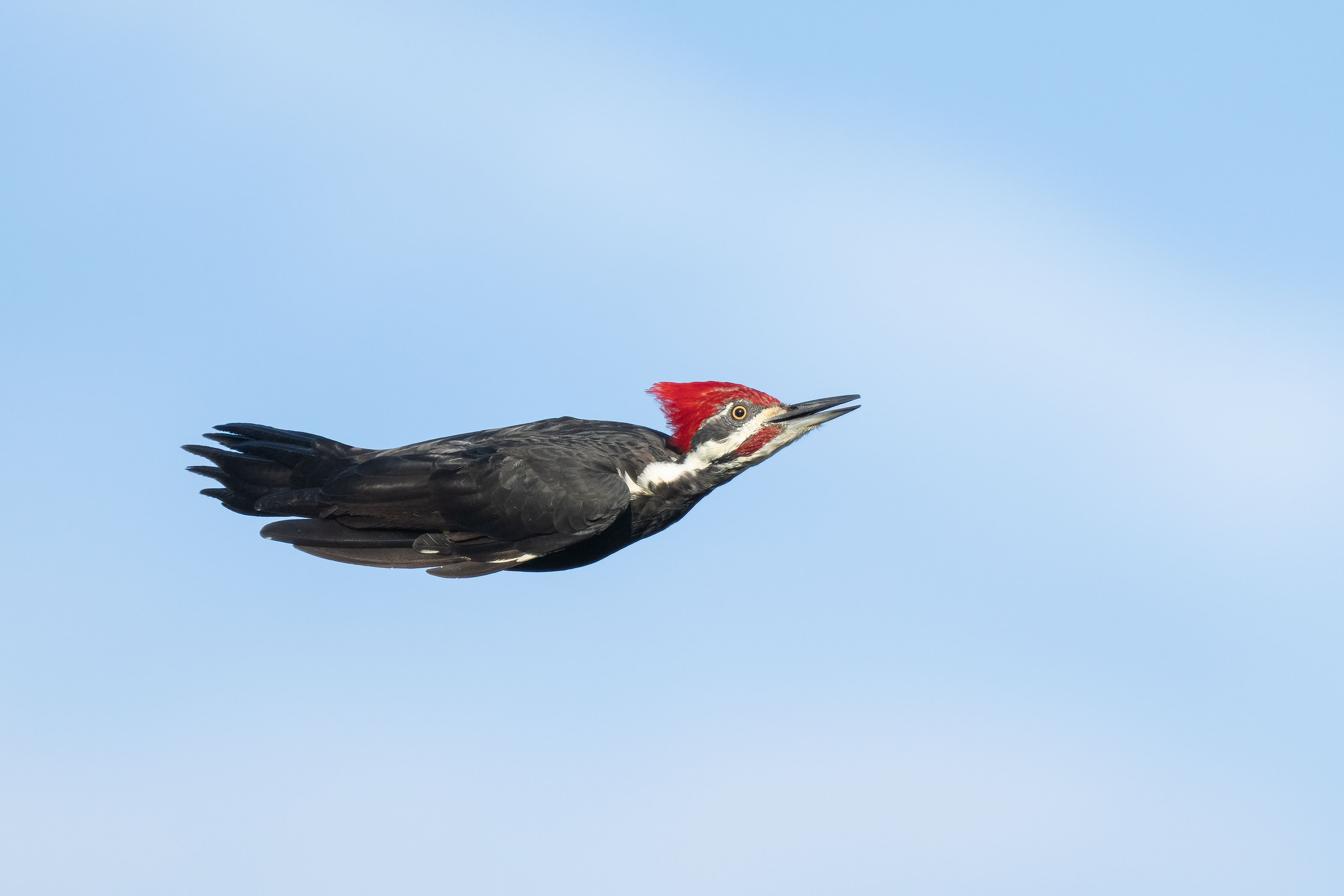This landscape photograph captures a striking bird mid-flight against a mostly blue sky with hints of white, feathery clouds. The bird, central to the image and flying from left to right, showcases a unique profile with a yellow eye and a slightly open, long, black beak. Its head is adorned with a red, mohawk-like crest that tapers to a triangular point, while its face features bold black and white stripes, accented by a touch of red beneath the beak. The bird's predominantly black body and contrasting white neck stripe make for a captivating view. The photograph's clarity and composition highlight the impressive details of the bird's vibrant head and sleek black feathers, creating a dynamic moment frozen in time.